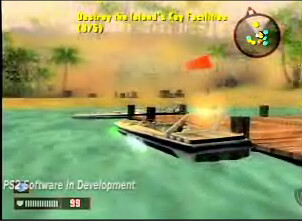In the image, which appears to be a screenshot from a video game in development for PS2, we see a vibrant scene featuring a greenish body of water with a wooden dock situated prominently on the left-hand side. Moored at this dock are two speedboats, one viewed from the side and the other from the back. The boat closest to the viewer is black and flies an orange flag. In the background, a sandy beach with lush green palm trees stretches across the horizon.

The screen is framed by various gaming interface elements. Across the top is blurred and illegible yellow text, including a command that begins with "destroy." The upper left corner features a circular minimap displaying the positions of players represented as yellow and green dots, roughly in equal numbers. On the lower left, there's a life bar accompanied by the number 99 in pink text, set against a dark green background with a heart icon to the left of the bar, indicating the player's health status.

An important note beneath these elements in white text reads "PS2 Software in Development." The image as a whole is a rectangular landscape orientation. The intricate details of the dock, speedboats, beach, and interface elements combine to create a dynamic and immersive game environment.